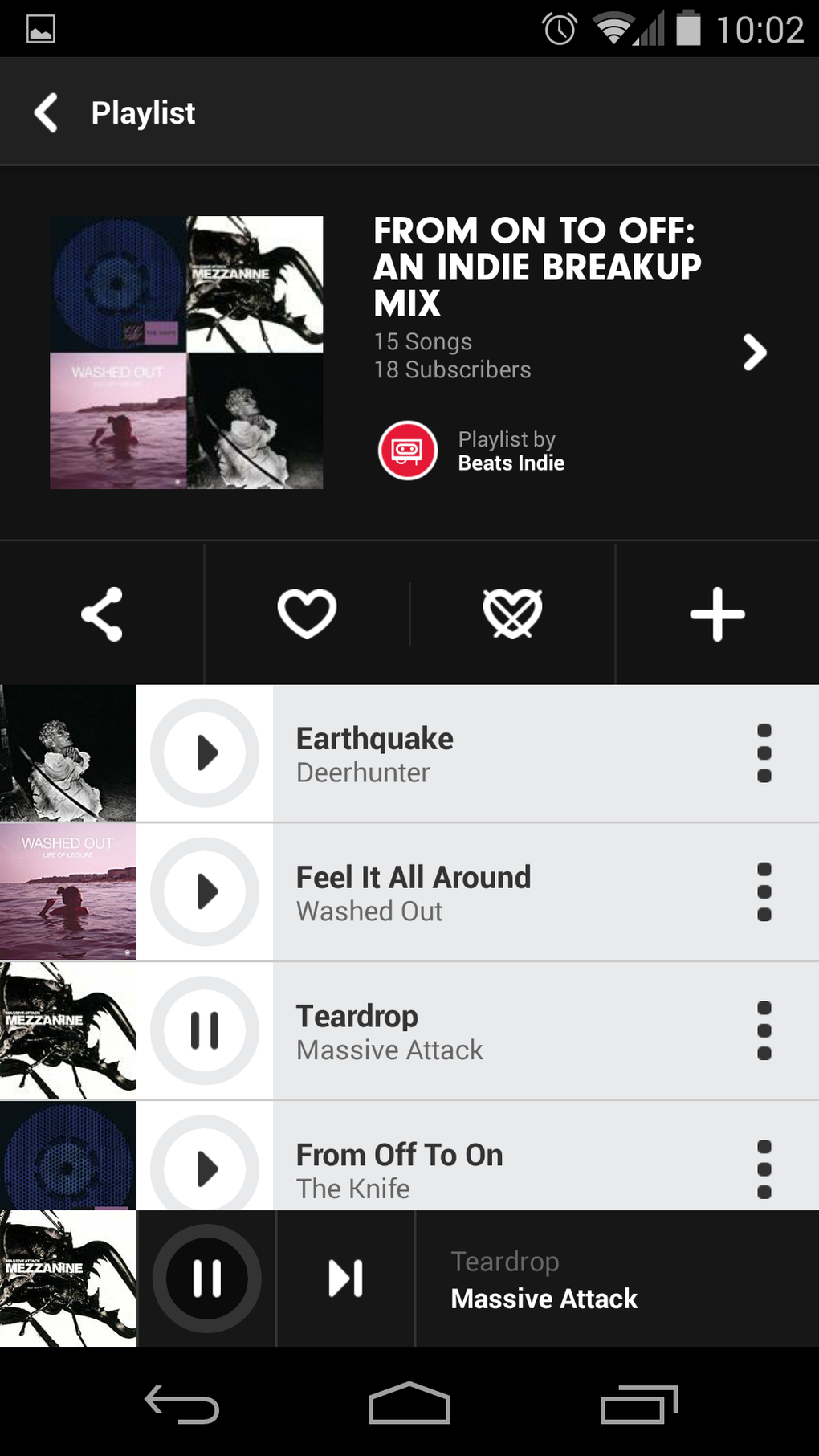Here is a cleaned-up and detailed caption for the described image:

---

A detailed view of a music app interface showcasing a playlist titled "From On to Off," an Indie breakup mix curated by Beats Indie. The playlist comprises 15 songs and has garnered 18 subscribers. Recognizable album covers from artists such as Deer Hunter and Massive Attack are prominently displayed. The cursor is currently on "Teardrop" by Massive Attack, indicating that it is the track being played. Other notable tracks in the playlist include "Earthquake" by Deer Hunter, "Feel It All Around" by Washed Out, and "From Off to On" by The Knife.

The app features a user-friendly design with individual track rows set against a light gray background, contrasting the black backdrop of the "Dark Months" section. Each track row includes functional buttons such as play/pause, share, like, and an option to add the track to a playlist. A back button is visible, presumably leading users to a larger music library. The phone's interface indicates a mostly full battery, suggesting ample listening time ahead.